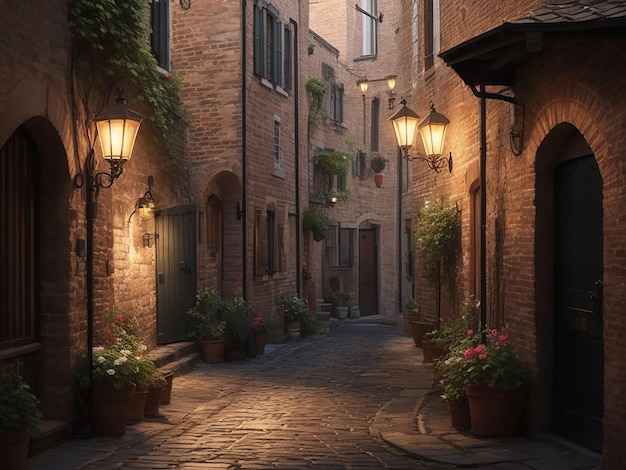The image captures a cozy evening scene of a winding cobblestone alleyway in a European village, presented in a landscape orientation. The alley is flanked by rows of brick and cobblestone townhouses, giving the area a residential feel. The narrow street gently curves to the right, disappearing around a corner, with a series of planters outside each doorway, featuring a mix of pink and white flowers. Street lanterns, with a coach-style design featuring black metal tops and white tapered bases, illuminate the scene brightly, casting a warm glow on the surroundings. The ground-level view accentuates the intricate details of the arched openings, partial balconies, and windows adorned with ivy and flowers. Amidst this picturesque setting, the ambiance suggests an old European city at night, bathed in lantern light that enhances the charming floral greenery outlined along the walkway.